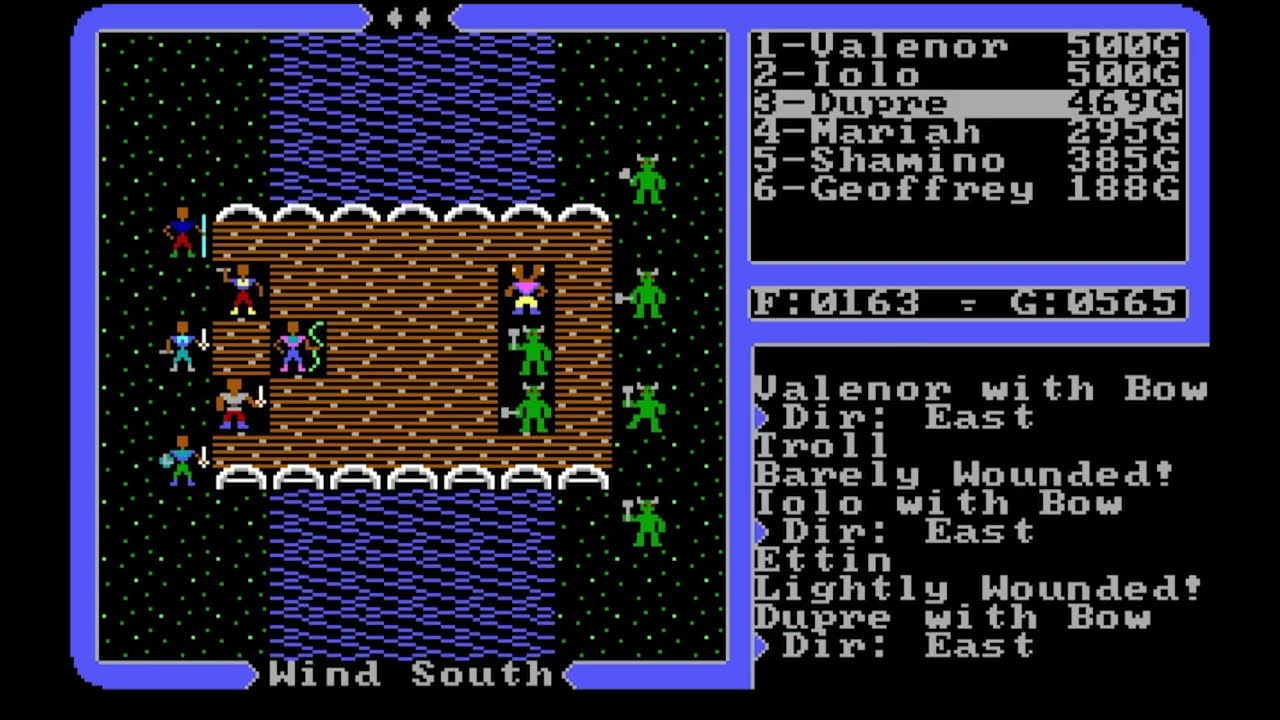This image is a screenshot from a retro, pixelated-style video game. The overall background is black, with an image slightly to the left bordered by blue lines. This bordered section showcases the game screen, which depicts a brown field or mud area populated by little figures resembling people, possibly engaged in combat or trying to navigate through the terrain. Opposing these figures are green monsters armed with hammers, suggesting a confrontation scenario.

The game screen is set against a space-like background, featuring small white stars and green dots scattered in the black expanse. There are blue sections above and below the brown field. Text at the bottom of the bordered image reads "Wind South" in white letters. On the right side of the screenshot, there is a table listing players' names and their scores or statuses: "1-Valinor 500g," "2-IOIO 500g," "3-Dupre 469g," among other similar entries. Beneath this table, more detailed textual information is provided about character positions and conditions, such as "Valinor with bow, Der East, Troll barely wounded," and similar descriptions for other characters like Aiolo and Dupre.